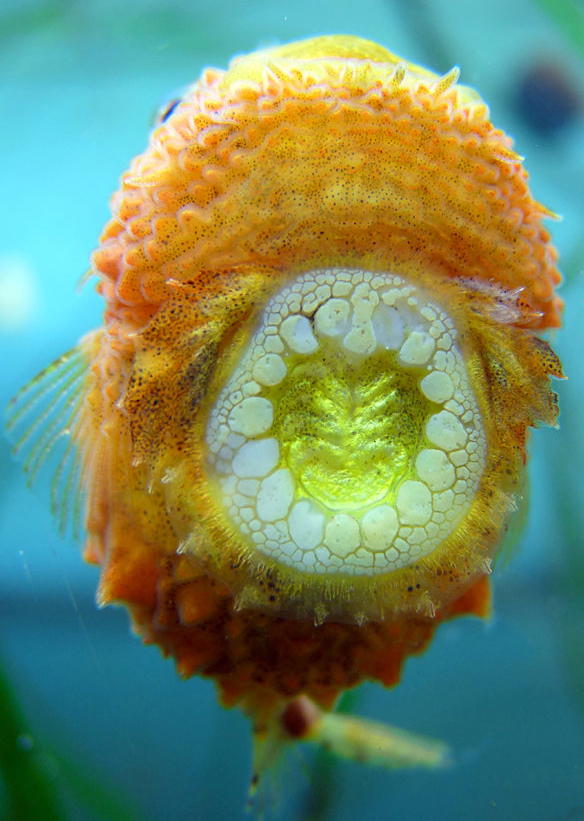This detailed color photograph captures the underside of a Pacific Spiny Lumpsucker, displaying its distinctive features against a backdrop of blue water. The fish is primarily orange with a bumpy, corally texture and an oval shape. On the left side, its translucent fin with green spines is visible. The fish's right eye barely peeks out from the upper left corner of the image. The most striking feature on its underside is a prominent circle in the middle, reminiscent of a suction cup. This circle has a bright yellow center, bordered by white that appears composed of small circles or cells, giving it a gelatinous look. Additionally, the fish's rear fins are yellow with black spots. Hints of plant life can be seen in the blue background, enhancing the aquatic setting.